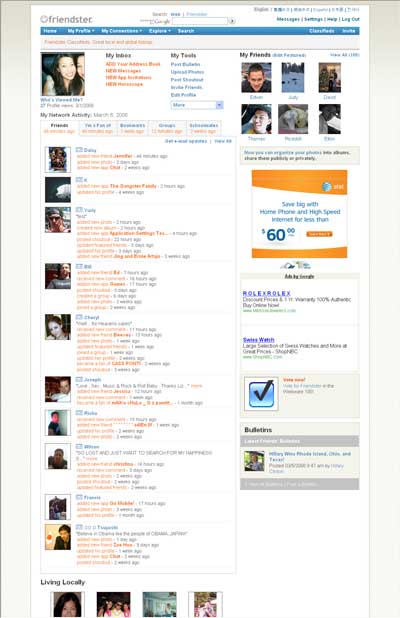This image is a minimized screenshot capturing a lengthy Friendster page, presented in a vertically-oriented, rectangular format with a centered alignment on a grey background. The Friendster page itself features a white background. Prominently, the Friendster logo is positioned in the top left corner.

Running vertically along the entire left side are numerous thumbnail images. Adjacent to these, on the right, are user bios. An AT&T square advertisement appears towards the right side, accompanied by a few smaller text ads located just below it.

At the very bottom of the page, there's a section titled "Living Locally," featuring four thumbnail images aligned horizontally. The image is cropped, cutting off the bottom halves of these thumbnails and the rest of the page.